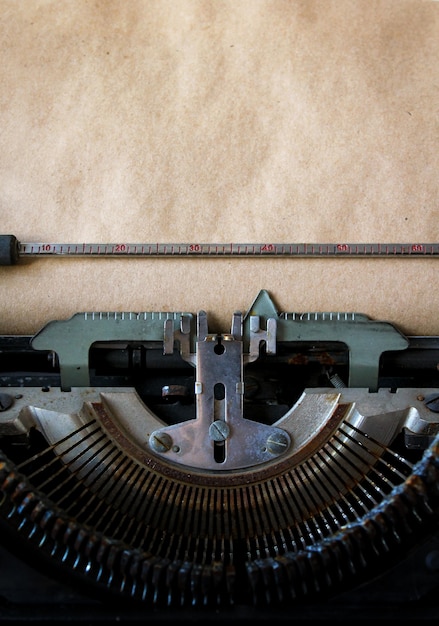The image is an extreme close-up color photograph of a typewriter, focusing on the metal mechanism used for measuring and spacing the paper. The upper portion of the image shows a weathered, pale brown piece of paper, resembling parchment, inserted into the typewriter. A thin, lined metal ruler bisects this paper, featuring numbers in red ink at regular intervals, starting from 10 on the left and extending to 60 on the right. The central and lower parts of the image reveal the intricate workings of the typewriter, specifically a half circular row of metal teeth and a green arrow pointing to the ruler. The metal parts of the device display shades of silver, brown, and a greenish hue, with the bottom fading to a dark black. The photograph does not include any visible letters, the keyboard, people, writing, or animals.